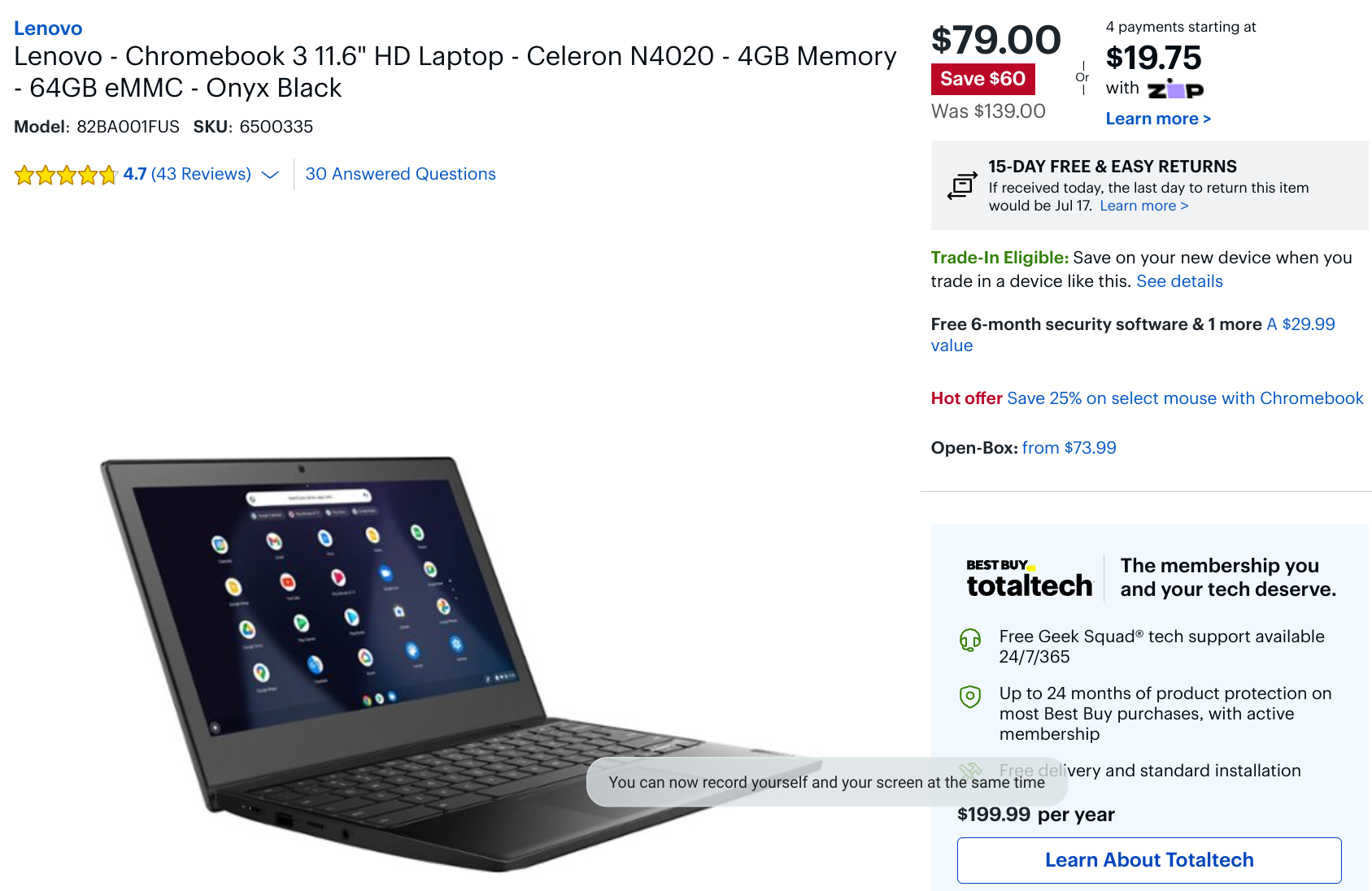**Detailed Caption:**

This image features an advertisement for the Lenovo Chromebook 3, a sleek and budget-friendly laptop designed for everyday use. The laptop boasts a compact 11.6-inch HD display and is powered by an Intel Celeron N4020 processor. It comes equipped with 4GB of memory and 64GB of eMMC storage, all encased in a stylish Onyx Black finish. The model number for this particular device is 82BA001FUS, and the SKU is 6500335.

In the image, the Chromebook is displayed in an open position, showcasing its neat and functional keyboard and screen. A standout feature highlighted in the advertisement is its capability to record both yourself and your screen simultaneously, enhancing the user experience for online meetings, tutorials, and more.

The laptop is currently available for a promotional price of $79, which is a significant saving of $60 from its original price of $139. Customers have the option to make this purchase in four interest-free payments of $19.75 via Zip. Additionally, the product is eligible for trade-in, providing even more value to prospective buyers. The advertisement also notes that the Lenovo Chromebook 3 has garnered a perfect 5-star rating, reflecting high customer satisfaction. For more information, viewers are encouraged to click on a 'Learn More' link.